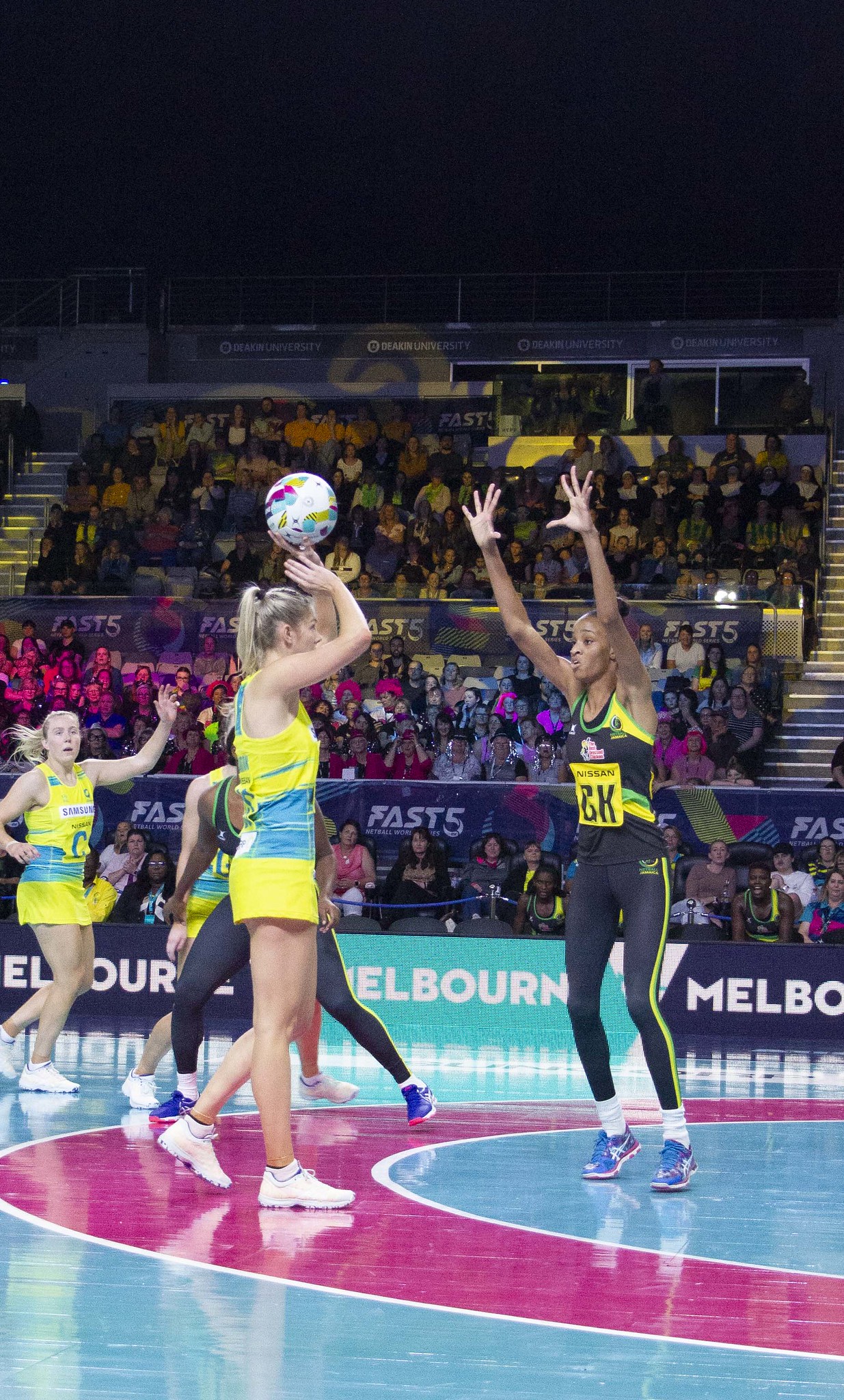The image captures an intense moment of a basketball game in Australia, specifically in Melbourne, as denoted by the repeated 'Melbourne' signage on the electronic billboard surrounding the stadium. The background showcases packed bleachers with fans, segmented by dark blue, aqua, and dark blue bands. There are also distinct lighting effects suggesting pinkish and yellowish hues among the spectators.

In the foreground, two prominent players are depicted: a blonde woman with a ponytail, wearing a yellow jersey and white tennis shoes, is holding a multicolored basketball above her head, preparing to make a pass or a shot. Defending her is a darker-skinned woman in a dark uniform with a yellow patch, raising her hands in an attempt to block. A closer look reveals another blonde woman in yellow, positioned behind the player with the ball, seemingly ready to receive a pass. Additionally, there's another player behind the woman with the ball, clad in a dark uniform, though her face isn’t visible in the image. The court’s floor features pink and blue hues, enhancing the visual dynamics of the scene.